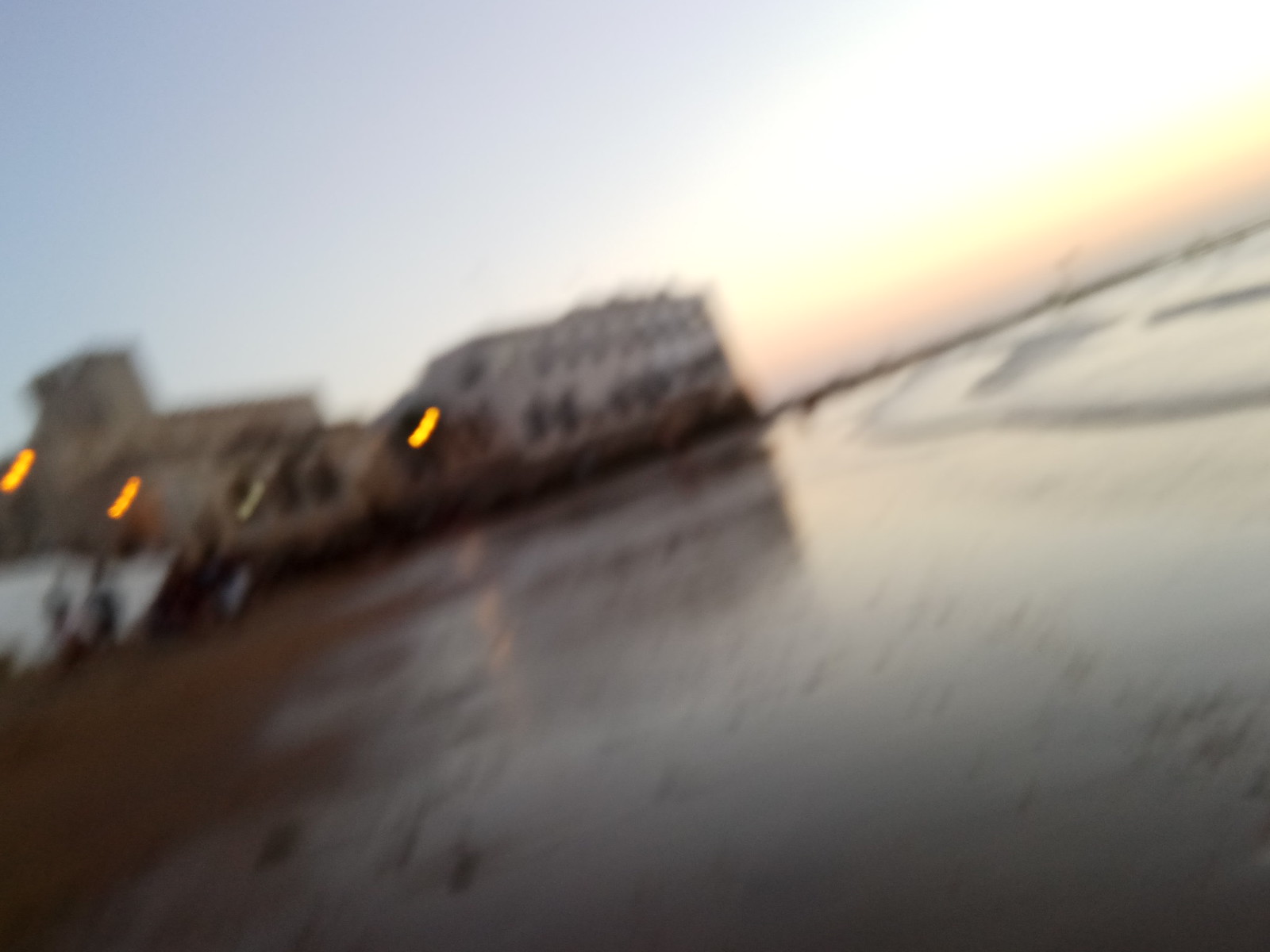This blurry and tilted photo captures a beachfront scene, likely taken around sunset, given the darkening sky with hues of orange, yellow, and light green. The image features an ocean with small waves gently lapping the sand. In the center are two large structures: a white, two-story rectangular building with numerous windows and a three-story brownish building resembling a step pyramid. The beach area includes a few scattered rocks, and a driveway or parking lot appears empty in the foreground. Though the picture is shaky and unclear, it evokes a vacation setting, possibly in Italy or Spain, with a medieval ambiance suggested by the architectural styles.